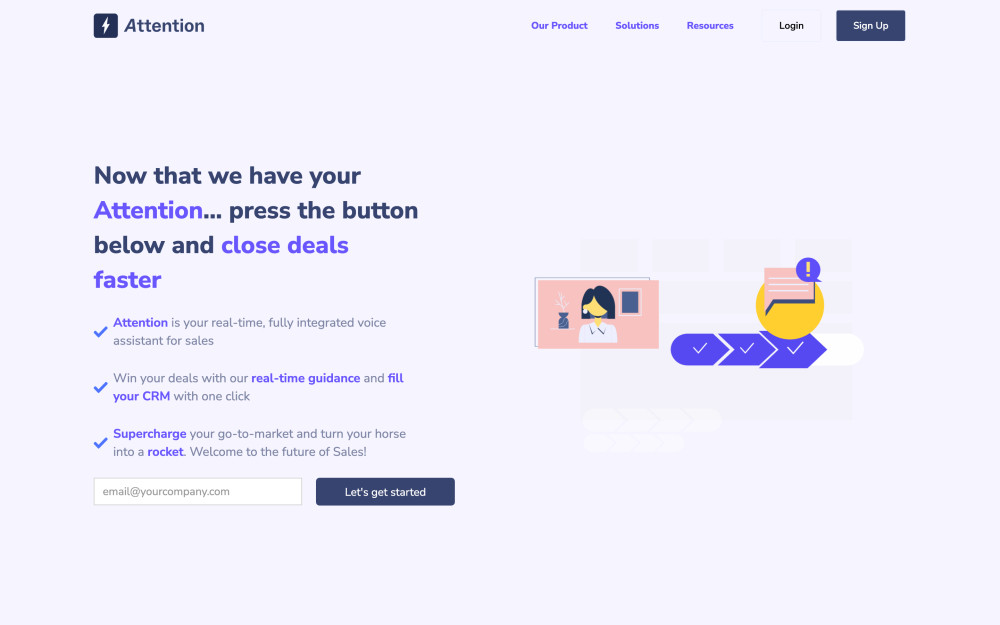The image depicts a promotional webpage for a company called "Attention," which features a lightning bolt as its logo. The tagline prominently displayed is, "Now that we have your attention," with the word "attention" highlighted in purple text. Below the tagline, there's an encouragement to "press the button below," emphasizing that "closed deals happen faster" also in purple text.

The bottom section of the webpage maintains a visual contrast with purple and gray text, outlining further details and accompanied by small blue check marks for emphasis. Users are prompted to enter their company email and click "Let's Get Started" to proceed with the sign-up process and explore the company's offerings.

To the right of the text, there is a graphic resembling a postcard, adorned with three purple check marks and a chat bubble featuring an exclamation point. The overall focus of the company "Attention" is on enhancing your sales processes and assisting with closing deals more efficiently.